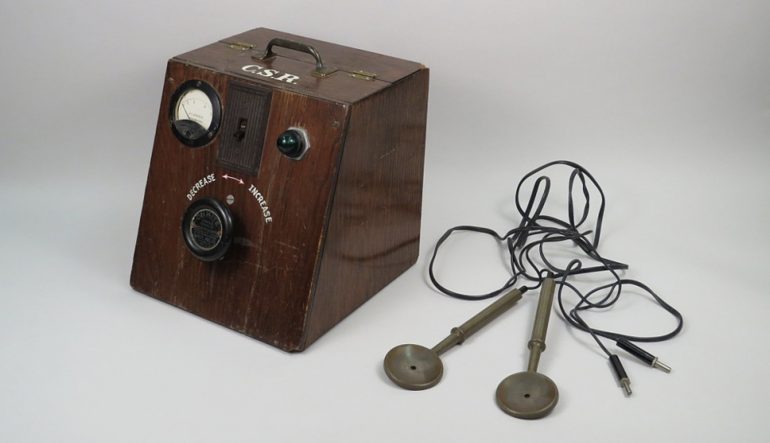This photograph showcases an antique wooden measurement device, possibly a defibrillator or a piece of maritime equipment. The equipment is housed in a medium to dark brown, trapezoidal wooden box that exhibits a shiny finish. The front face of the box slopes downward from top to bottom. At the top is a metal handle, and the letters "CSR" (possibly the manufacturer's initials) are visible.

The front panel features several controls and indicators:
- A central black dial with white text reading "decrease" to the left, "increase" to the right, and a white arrow in between.
- Directly below the text is a switch that resembles a light switch.
- To the left, there is a white gauge with a visible needle, though the numbers are indistinguishable.
- Up and to the right of the black dial is a small knob and a green light.
- Attached to the right side of the device are two circular paddles with long, thin handles. These paddles have black wires that terminate in plugs resembling 3.5 mm jacks.

The device’s condition and design elements, including metal hinges and a door on top, point to its antique nature, possibly used for measurements or early medical applications. The background of the image is light gray, which contrasts with the dark, polished look of the wooden box.